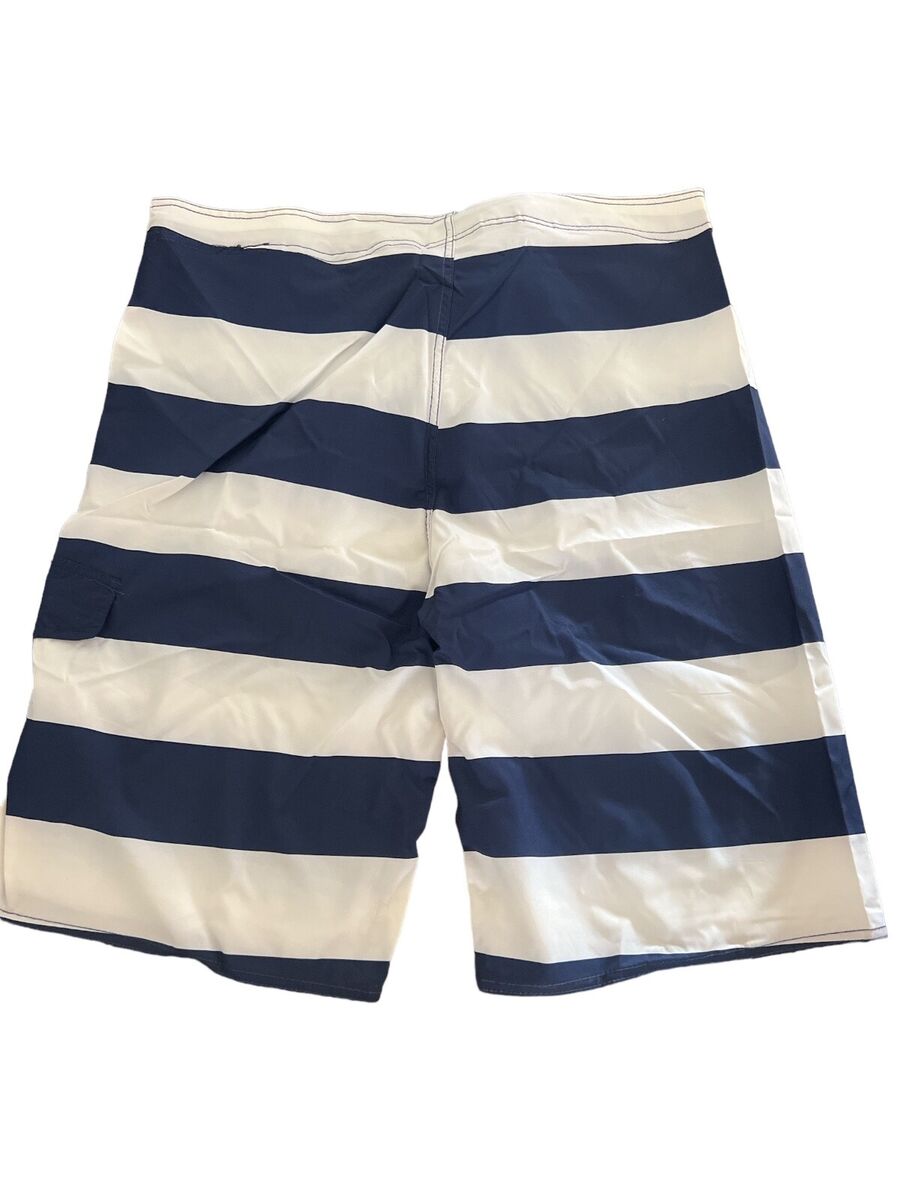This detailed photo features a pair of boys' swim shorts displayed against a pristine white background. The shorts, primarily composed of alternating navy blue and white stripes, exhibit a slightly wrinkled texture, particularly noticeable where they have been folded across the legs. Each stripe is of equal width except for the very top and bottom ones, which are marginally shorter. The top features a white stripe, followed by a series of alternating navy blue and white stripes extending down the length of the shorts. Notably, there is detailed double stitching at the top, with a navy stitch on the white stripes and a white stitch on the navy stripes, creating a contrasting pattern throughout. These board shorts are designed without a tie, zipper, or pockets, adding to their streamlined appearance.